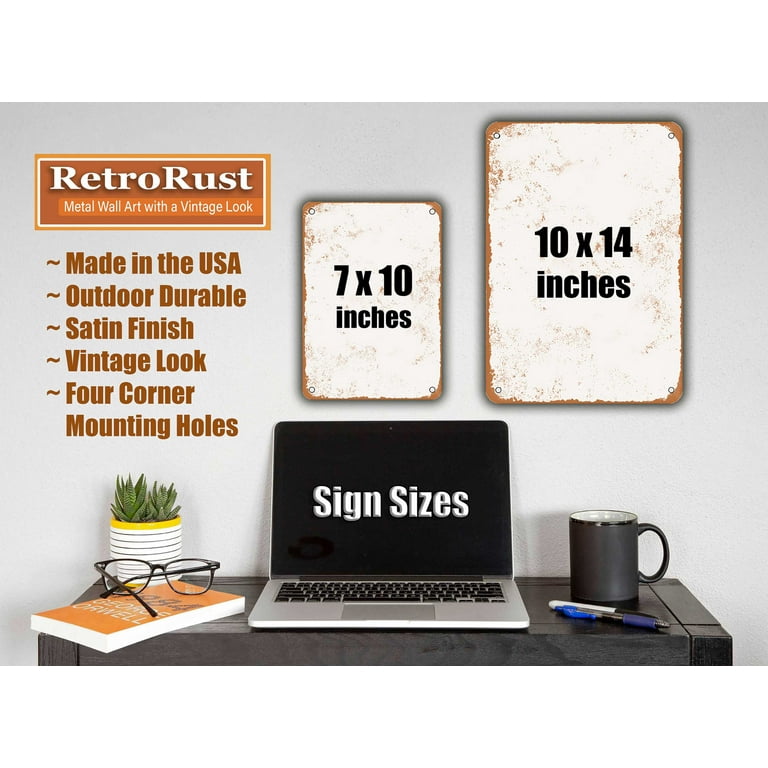The composite image showcases a desk setup prominently featuring advertising for "Retro Rust" metal wall art with a vintage look. Against a white background, the upper right section of the image displays two worn, white posters with brown splotches and an orange outline—one measuring 10 by 14 inches and the other 7 by 10 inches. Both posters have their dimensions labeled in the center. An orange banner at the top left reads "Retro Rust" in white text, followed by bullet points in brown text indicating features: "Made in the USA, Outdoor Durable, Satin Finish, Vintage Look, Four Corners, Mounting Holes."

Beneath this, on a black painted wooden table, several objects are neatly arranged. The centerpiece is an open silver laptop with a black screen that displays the text "sign sizes." Positioned around the laptop are various items: a black mug at the back right, two pens (a Sharpie and an ink pen) at the bottom right, and an orange book titled "1984" by George Orwell at the bottom left. Resting atop the book is a pair of black-rimmed glasses. Behind the book, a white plant pot with yellow and black stripes houses a succulent with pointy green leaves, possibly a small aloe plant. The composition highlights the desk’s tidy appearance while emphasizing the featured vintage wall art.